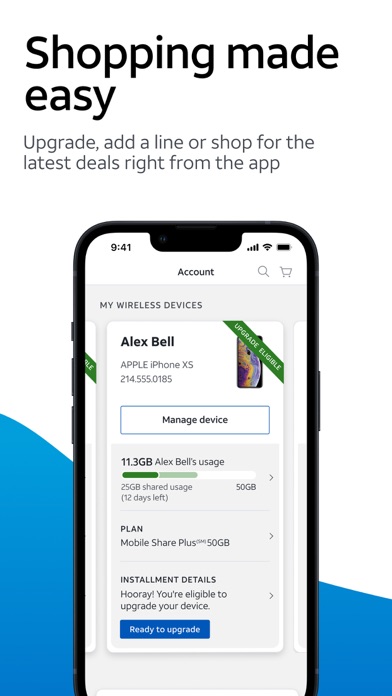This screenshot features a predominantly white background, save for a blue section that occupies the bottom portion of the image, rising nearly halfway up the left side before sloping downward to the right. At the top, large, bold black letters prominently proclaim "Shopping Made Easy." Two lines below this, in gray text, it reads, "Upgrade, add a line, or shop for the latest deals right from the app."

Approximately four lines beneath this text, centered within the image, is a depiction of a smartphone. On the screen of the smartphone, the word "Account" appears at the top in black text. Below this, it reads "My Wireless Devices." Further down, positioned within a white and gray rectangular box, the name "Alex Bell" is boldly written in the upper left-hand corner in black. To the right, there's an image, partially obscured by a green banner across the top-right corner.

Below this section is a button framed in blue, labeled "Manage Device." Underneath this button is a gray segmented box with three distinct parts. The first segment displays "11.3 GB Alex Bell's Usage," accompanied by a green and white status bar indicating data consumption. Below the usage information, details about the plan are provided, followed by a section detailing installment information.